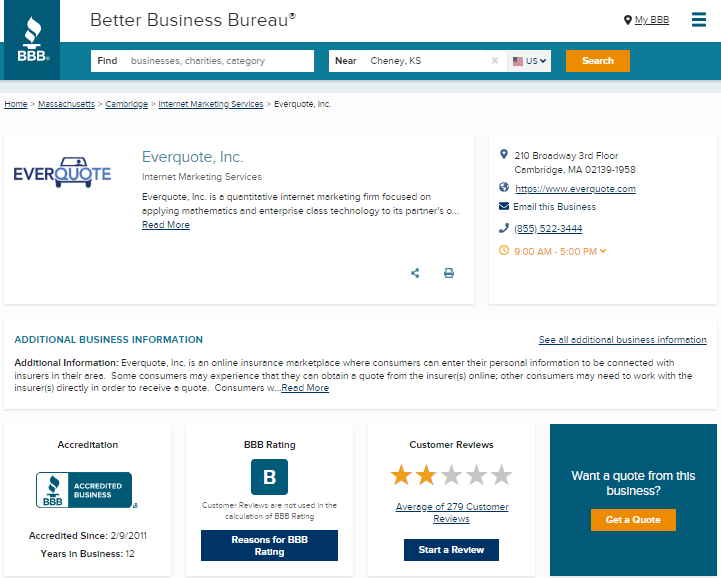Detailed Caption: 

The image depicts a webpage set to the Better Business Bureau (BBB) platform. In the upper left corner, the traditional BBB logo, featuring a torch, is prominently displayed on a blue background. Adjacent to the logo, the text "Better Business Bureau" is clearly visible. At the top of the webpage, it also reads "MyBBB," indicating a personalized section of the site. 

Below these headings are two search bars designed to assist users in finding relevant information. The first search bar, labeled "Find," allows users to search for businesses, charities, or categories. The second search bar is labeled "Near" and is currently set to "Cheney, KS, U.S.," suggesting the location can be modified. Additionally, there is a conspicuous yellow search button that users can click to initiate their search. The website interface seems user-friendly and functional for looking up specific businesses or services efficiently.